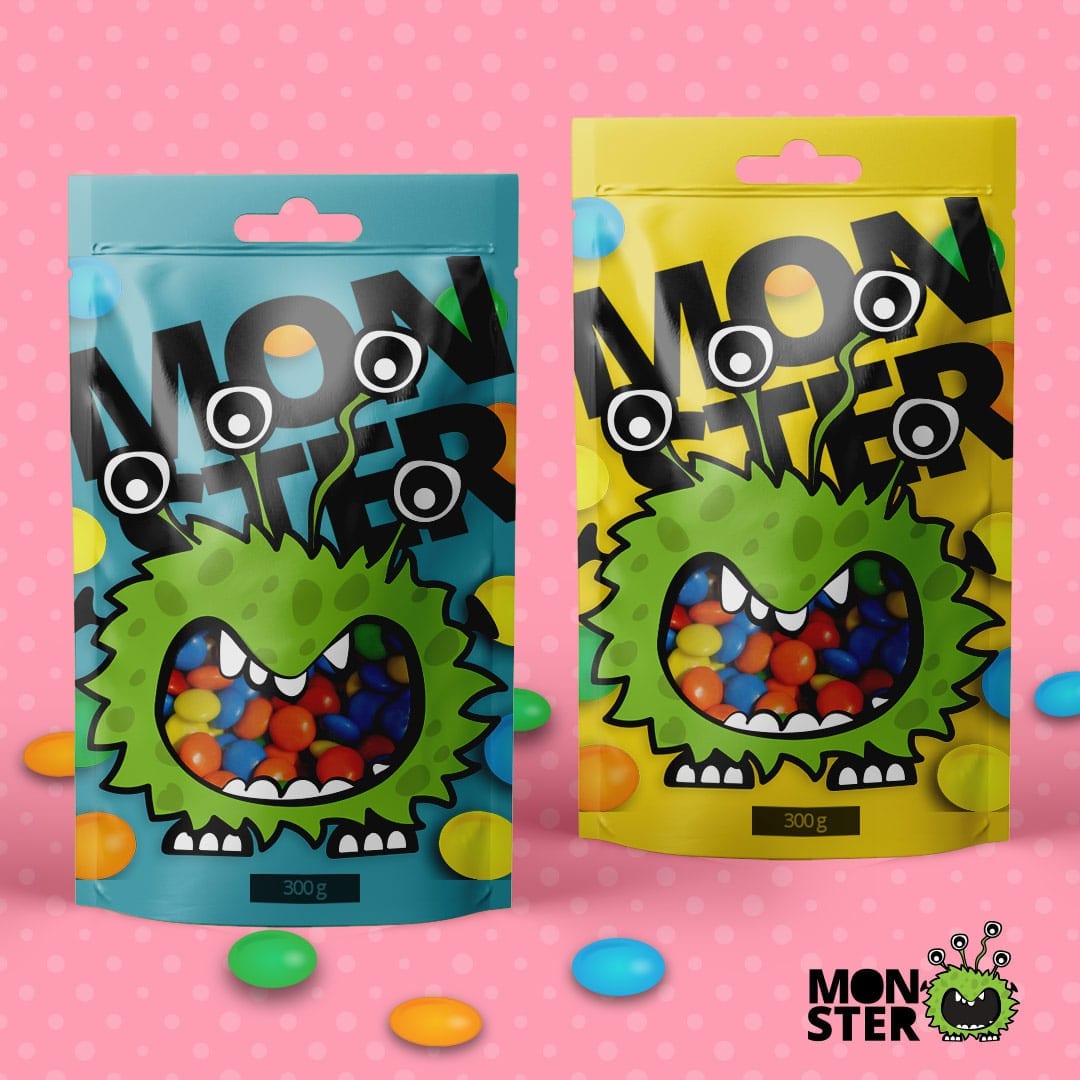In the image, two vibrant bags of candy stand against a pink polka-dotted backdrop. The bags, one light blue and the other light yellow, each feature a whimsical green monster with dark green spots, a wide-open mouth displaying teeth, and four quirky eyes atop tendrils. The front of the bags prominently displays the brand name "Monster," with the letters M-O-N across the top and S-T-E-R below. Clear windows in the packaging reveal colorful candies within. At the bottom of each package, it is noted that the content weighs 300 grams. Scattered around the bags on the pink-dotted surface are brightly colored candies. In the lower right corner of the image, the word "Monster" is written again, accompanied by the same alien logo from the package, enhancing the playful and inviting advertisement.